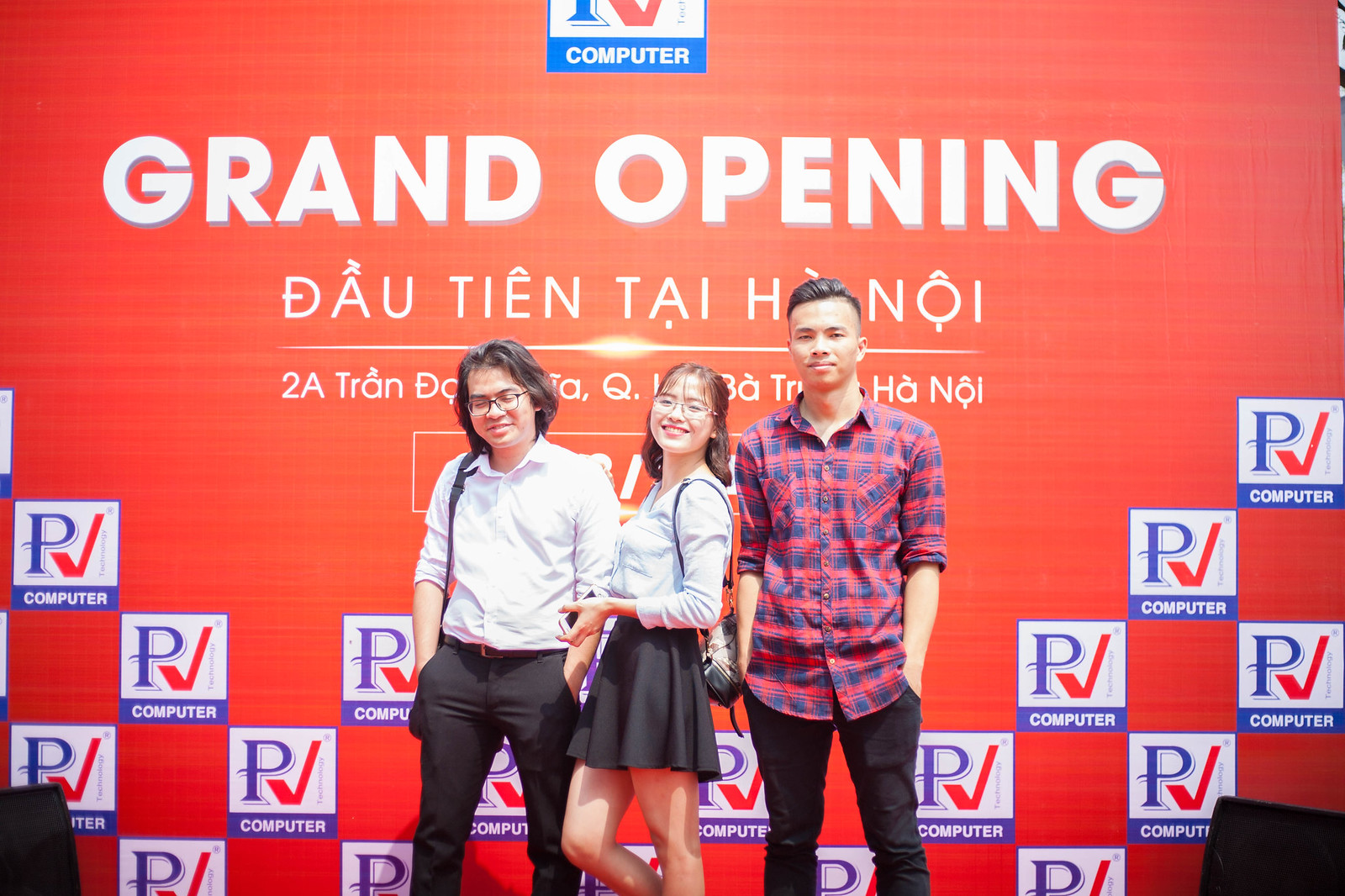In this photo, three young Asian individuals—a man on the left, a woman in the center, and another man on the right—are standing in front of a grand opening banner for P-CHECK COMPUTER. The backdrop is predominantly red, though it features repeating white squares with blue and orange accents, displaying the company's logo: a letter "P" with a check mark, followed by the word "computers." The central woman is smiling, wearing a white blouse, a black skirt, and glasses, and she is holding a black purse. The man on her right has on a red and blue checkered shirt with gray pants. The man on the left is dressed in a light blue (almost white) shirt, with a strap over his right shoulder, and dark gray trousers. Both men are also smiling at the camera. Above them, text in both English and a foreign language reads "Grand Opening."